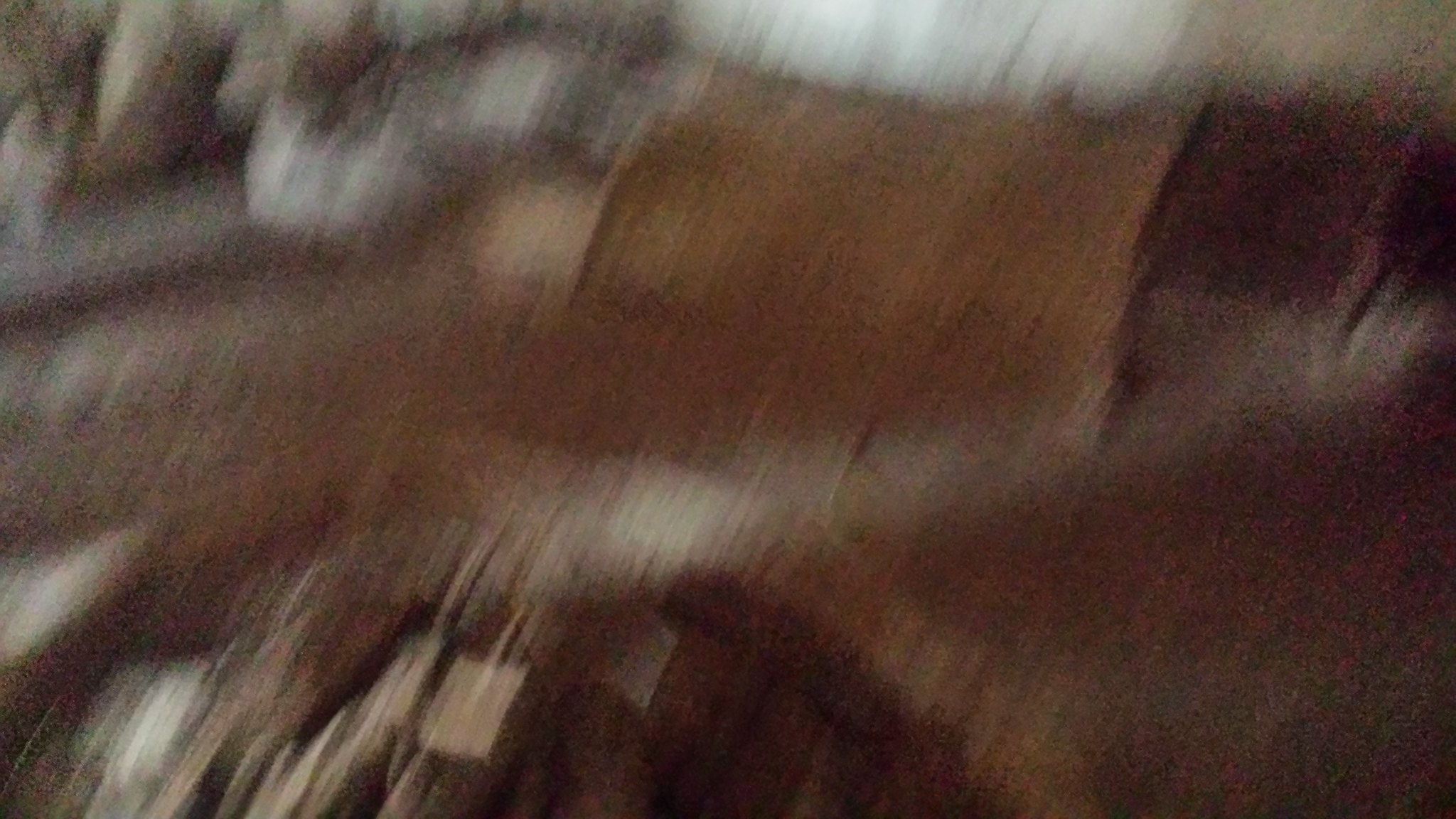This image is of extremely poor quality, with visual elements streaked and blurred together, making it difficult to decipher. In the upper left corner, there appears to be a burlap-type bag or something resembling it. The middle section of the image features a light tan color interspersed with darker brown hues on the right side. A prominent white streak cuts horizontally across the middle. The top portion of the photo is dominated by a solid white area, while the bottom exhibits a rounded form that suggests the presence of people, possibly wearing tan-colored clothing, although this is uncertain.